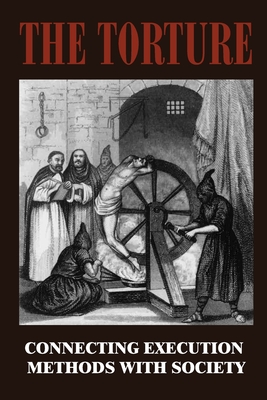The cover of the book titled "The Torture" features an intense and dramatic black and white drawing set against a black background. At the top of the cover, the title "The Torture" is prominently displayed in large, bold red text. Below, in white text, the subtitle reads, "Connecting Execution Methods with Society." The focal point of the illustration depicts a harrowing scene: a naked man, save for a loincloth, is bound to a large wheel with his back arched in extreme discomfort. His arms are tied behind him, and his legs are secured to the wheel. The man looks upwards, possibly in anguish or despair. 

Two hooded figures, dressed in black robes, are positioned beside the wheel. The figure on the right is standing and operating a crank that likely turns the wheel, while the figure on the left crouches and seems to be stoking a fire beneath the wheel with an accordion-style fan. In the background, three men appear to be observing the scene, engaged in what looks like a discussion. The setting and attire of the figures evoke a medieval or inquisitorial atmosphere, further emphasizing the grim and torturous nature of the scene.